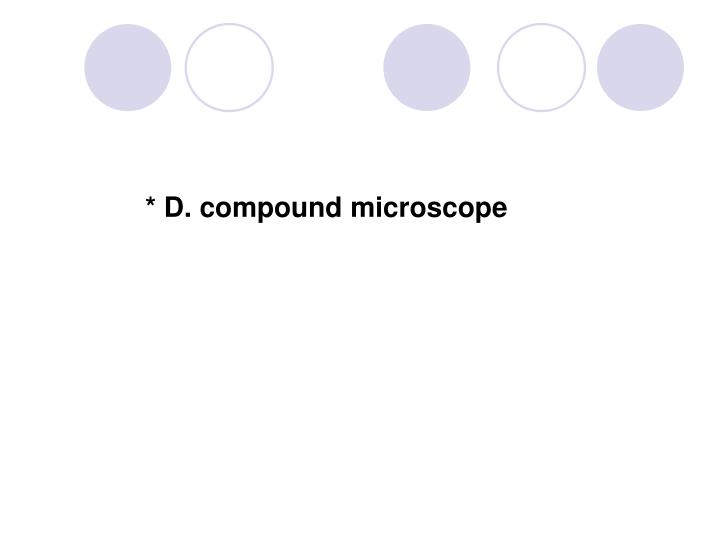The image features a pure white background with a centrally-aligned block of text and a row of five circles near the top. The text, bold and in a standard font, reads: "☆ Decompound Microscope." The arrangement places emphasis on the capital "D" followed by "compound microscope" in lowercase. 

Above the text, the circles are divided into two groups. On the left, there are two circles: a light blue filled circle followed by a white circle with a light blue border. To the right, separated by slightly larger spaces, there are three circles arranged in disc-circle-disc pattern: a light blue filled circle, another white circle with a light blue border, and another light blue filled circle. This evenly spaced arrangement is set against the blank expanse of the background, lending a clean, minimalist aesthetic. The placement and style suggest that this image might be part of an educational or scientific presentation slide.